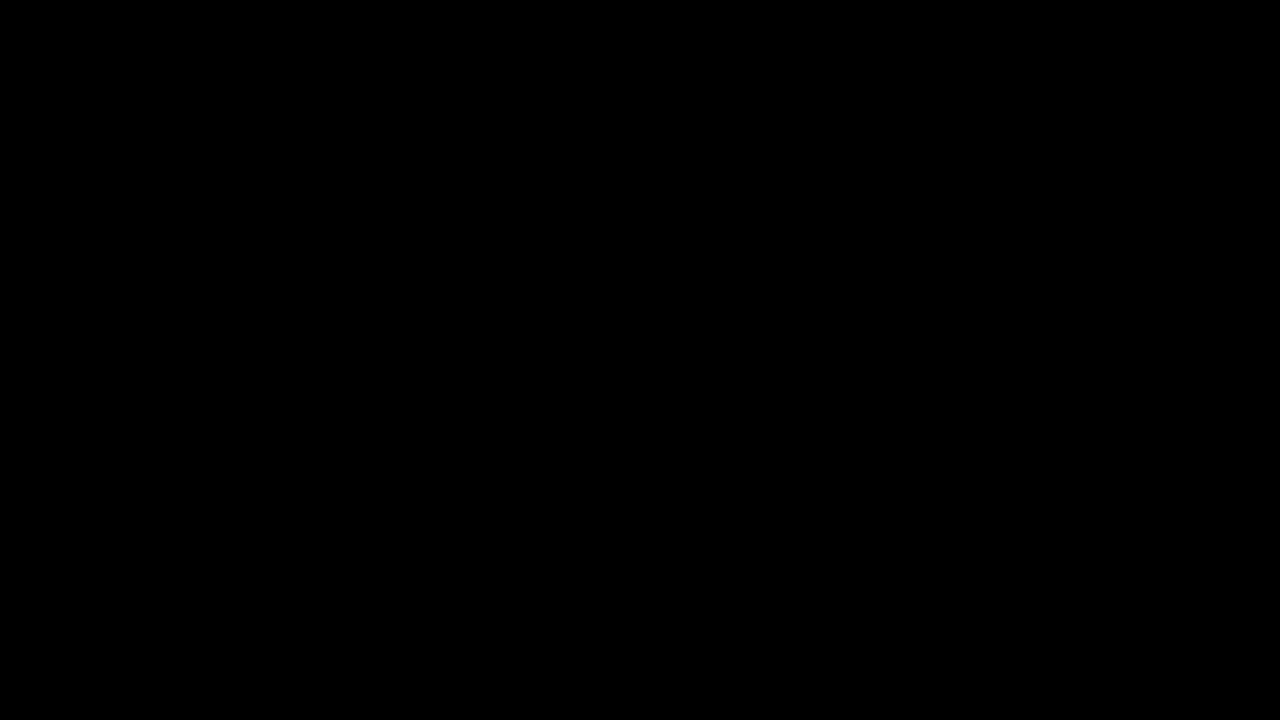The image depicts a large, horizontal, matte black rectangle with sharp, defined corners. The rectangle is oriented in landscape format, where its width is greater than its height. The color is a deep, solid black with no gradations, shading, or text anywhere on the image. There are no ambient shadows, afterimages, or any other distinguishing features—just the unvarying, uniform blackness. The stark simplicity of the rectangle suggests it could potentially serve as a digital background for future artwork or another purpose, though presently, it remains a pure black rectangle against the white background.